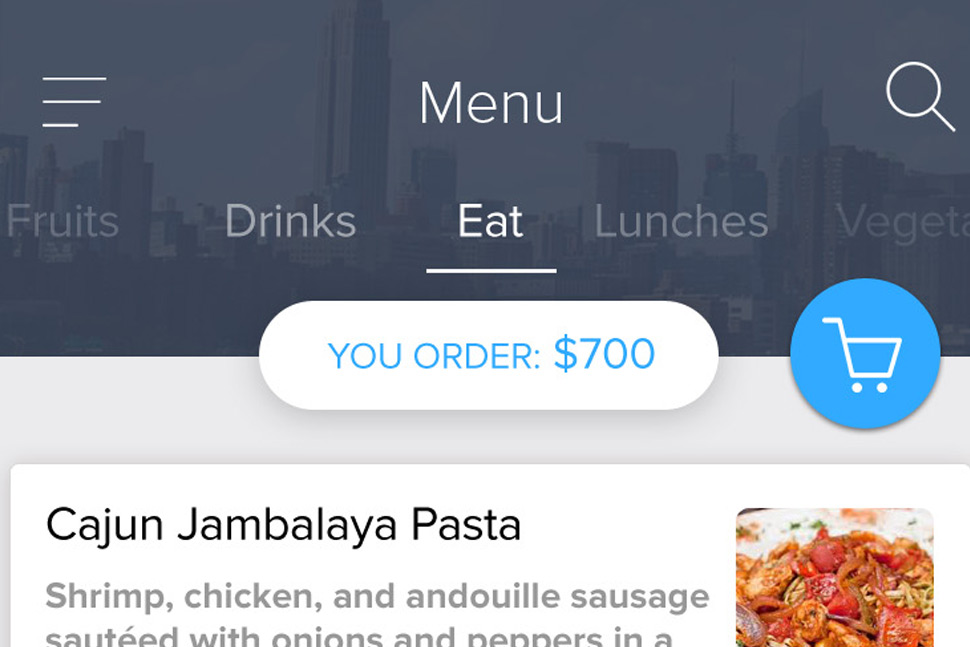The image depicts a modern web page with a layout approximately 20-30% wider than it is tall, providing a sleek and efficient user interface. 

At the top of the webpage, a semi-transparent, gray overlay partially obscures a faint cityscape filled with towering commercial buildings, giving a sophisticated urban ambiance. On the upper left corner, three stacked lines signify a menu icon, labeled "menu." Centrally placed in white text is the website's title, flanked on the right by a search icon represented by a magnifying glass.

Below this header, a horizontal navigation bar in light gray text lists various categories: "Fruits," "Drinks," "Eat" (highlighted in white with an underline to indicate the current selection), "Lunches," and a truncated category labeled "V-E-G-E-T."

Further down, an elongated blue oval features the text "Your Order: $700" in bold, blue lettering. Adjacent to this, a teal circle houses a white shopping cart icon, likely linking to the user's cart.

The main content section has a clean white background, displaying a prominent dish named "Cajun Jambalaya Pasta" in striking black text. To the right of this label is an appetizing image of the meal, and below it, a list of ingredients is subtly presented in gray text, detailing the delicious components of the featured dish.